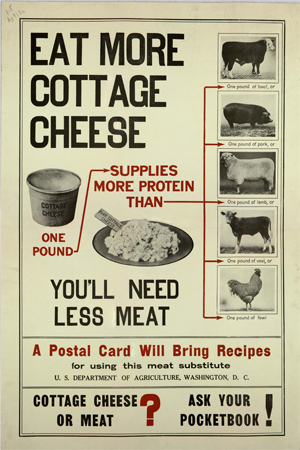The image is an aged poster from the U.S. Department of Agriculture promoting cottage cheese as a high-protein alternative to meat, likely from the 1940s or '50s. The rectangular advertisement has an off-beige background with a black border. At the top left, bold black text reads, "Eat more cottage cheese." Below this text is an image of a one-pound tub of cottage cheese next to a black plate also featuring cottage cheese. Red text adjacent to this image asserts that cottage cheese "supplies more protein" than "one pound of meat" from five different types of livestock: a cow, a pig, a sheep, a calf, and a chicken, all depicted in descending order on the right-hand side. Additional black text states, "You'll need less meat," followed by a red line of text encouraging viewers to send a postal card to receive recipes for using cottage cheese as a meat substitute. This line reads, "A postal card will bring recipes for using this meat substitute," and is attributed to the "U.S. Department of Agriculture, Washington, D.C." At the bottom, the ad concludes with the slogan, "Cottage cheese or meat? Ask your pocketbook!" emphasizing cost-effectiveness and high protein content of cottage cheese. The poster combines red and black fonts to deliver its message clearly, aiming to persuade consumers to make a more economical and protein-rich choice during times of meat scarcity.